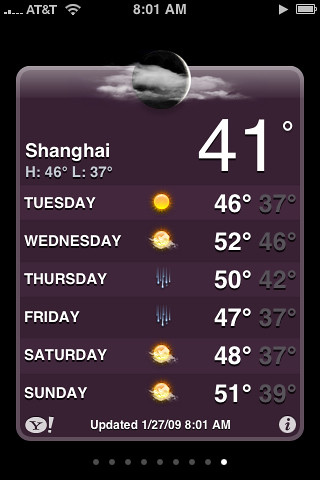The image appears to be a screenshot taken from a smartphone. In the top-left corner, two white bars indicate a mobile signal, followed by the text "AT&T" and a Wi-Fi icon. To the right of these, the time is displayed as 8:01 a.m. Continuing to the right, there is a playback button adjacent to a battery icon displaying its charge status.

The main content of the screenshot is a weather update set against a gray background. At the top, there is an icon depicting a moon obscured by clouds, indicating nighttime weather conditions. Beneath this, on the left, the location "Shanghai" is displayed, with the current temperature listed as 41°F. The forecast also includes the high for the day at 46°F and the low at 37°F.

Below this data, a weekly weather forecast extends from Tuesday through Sunday:

- **Tuesday**: Sunny icon with a high of 46°F and a low of 37°F.
- **Wednesday**: Partially cloudy icon with a high of 52°F and a low of 46°F.
- **Thursday**: Rain icon with a high of 50°F and a low of 42°F.
- **Friday**: Rain icon with a high of 47°F and a low of 37°F.
- **Saturday**: Partly cloudy icon with a high of 48°F and a low of 37°F.
- **Sunday**: Partly cloudy icon with a high of 51°F and a low of 39°F.

At the bottom of the screen, the Yahoo Weather app icon is present, with an update timestamp noting the data was refreshed at 8:09 a.m. on January 27th, 2009.